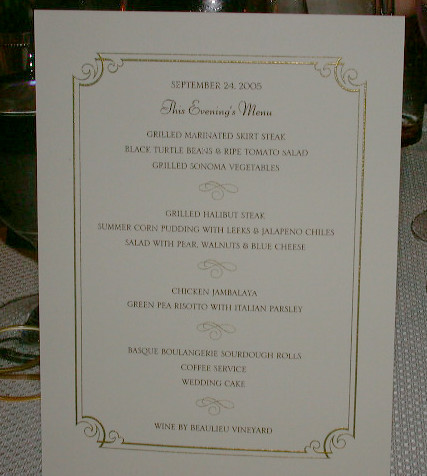This image showcases a formal wedding menu from September 24th, 2005. The menu is printed on thick, white cardstock with an elegant gold design framing the borders. The header reads "This Evening's Menu," and details an exquisite selection of dishes prepared for the occasion:

- **Grilled Marinated Skirt Steak**
- **Black Turtle Beans and Ripe Tomato Salad**
- **Grilled Sonoma Vegetables**
- **Grilled Halibut Steak**
- **Summer Corn Pudding with Leeks and Jalapeño Chilies**
- **Salad with Pear, Walnuts, and Blue Cheese**
- **Chicken Jambalaya**
- **Green Pea Risotto with Italian Parsley**
- **Basque Boulangerie Sourdough Rolls**
- **Coffee Service**
- **Wedding Cake**
- **Wine by Beaulieu Vineyard**

The carefully curated menu items suggest a highly personalized dining experience, likely selected during the RSVP process for the wedding.